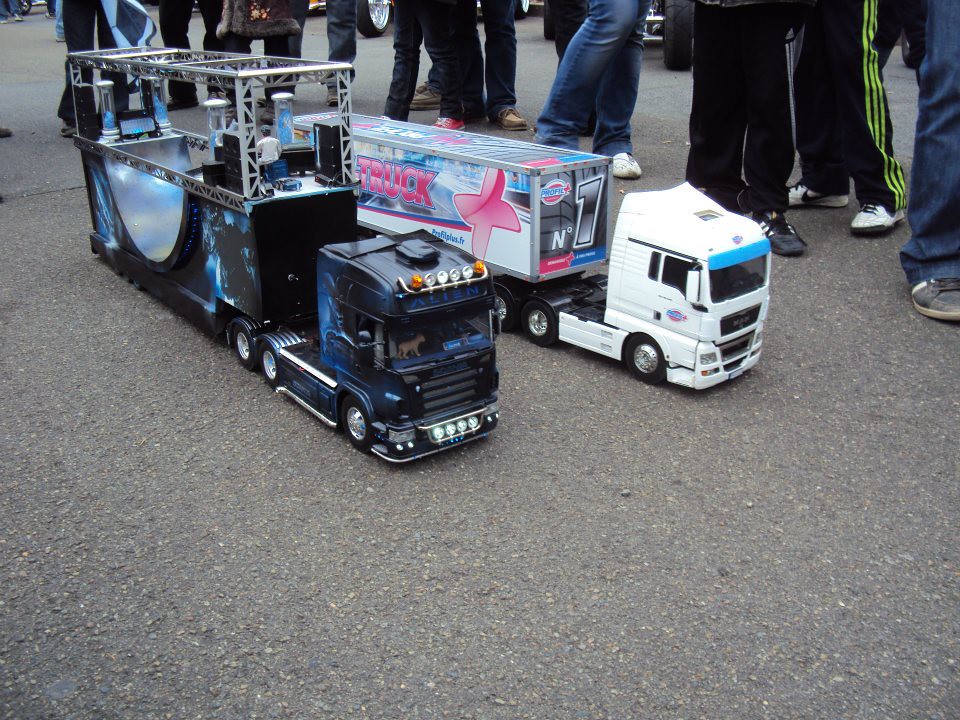In this outdoor photograph, two child-sized toy semi-trucks are positioned on a concrete surface, with a line of onlookers in long pants and running shoes visible in the background. The first truck is a dark blue or black color with intricate detailing, including a cab adorned with red, yellow, and white lights, and a beige toy dog visible through the front windshield. This truck tows an open-framed trailer, featuring a skate ramp and what appears to be a small DJ setup on top. The second truck, to the right, is white with a matching trailer that prominently displays a pink flower, the word "truck" in pink lettering, and the number one. The trucks' black tires and aluminum rims are clearly visible, and all elements are carefully scaled to child size.